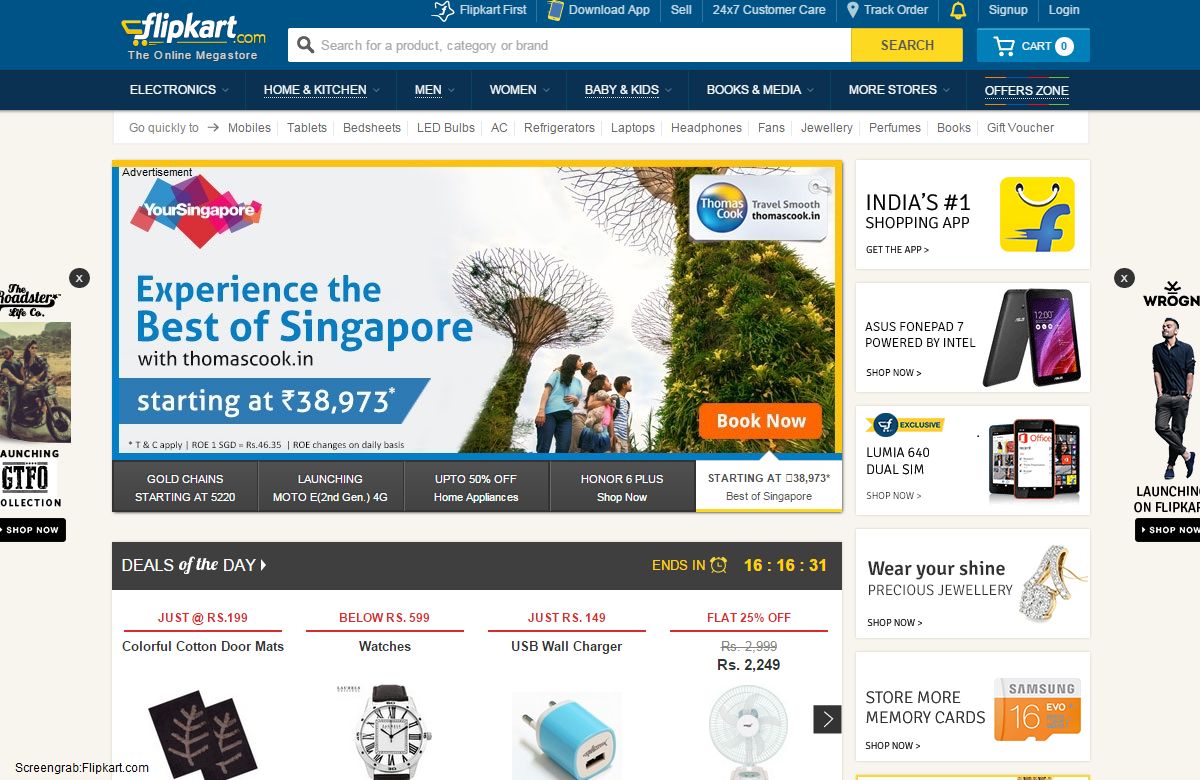**Detailed Caption:**

This screenshot captures the homepage of Flipkart, a prominent online mega store, buzzing with a plethora of categories and offers. At the very top of the page, a blue navigation bar prominently displays the Flipkart logo in white alongside the tagline "The Online Mega Store." This is followed by a search bar with a yellow search button and a blue cart icon indicating an empty cart.

Above the search bar, there are options including Flipkart First, Download, Upsell, 24-7 Customer Care, Track Order, Sign Up, and Log In. Directly below the main navigation bar, there's a secondary menu offering various categories such as Electronics, Home & Kitchen, Men, Women, Baby & Kids, Books, Media, More Stores, and Offer Zone.

Further down, quick links are available for popular items: Mobiles, Tablets, Bed Sheets, LED Bulbs, AC Refrigerators, Laptops, Headphones, Fans, Jewellery, Perfumes, Books, and Gift Vouchers.

The center of the screen features a large, vibrant advertisement with the tagline "Your Singapore" showcasing a kaleidoscopic logo reminiscent of multicolored faceted jewels or mountains. Accompanying the logo is a promotional offer: "Experience the best of Singapore with Thomascook.in, starting at ₹38,973." The ad includes a "Book Now" button on the right and an image of people admiring peculiar-shaped trees.

Below the central advertisement, the "Deals of the Day" section displays an assortment of discounted products including a watch, a plug, a fan, and some doormats.

To the right of the deals section, the webpage highlights that Flipkart is "India's Number One Shopping App", illustrated with an image of smartphones. Additional highlighted offers include "Wear Your Shine" and promotions for various memory cards.

The webpage is bordered with side banners; on the left, there's an image of a person riding a motorbike, while the right side features a man dressed in a dark top and black leather trousers.

Overall, the page is rich with visual stimuli and multiple sections designed to draw the shopper's attention to various deals and categories.